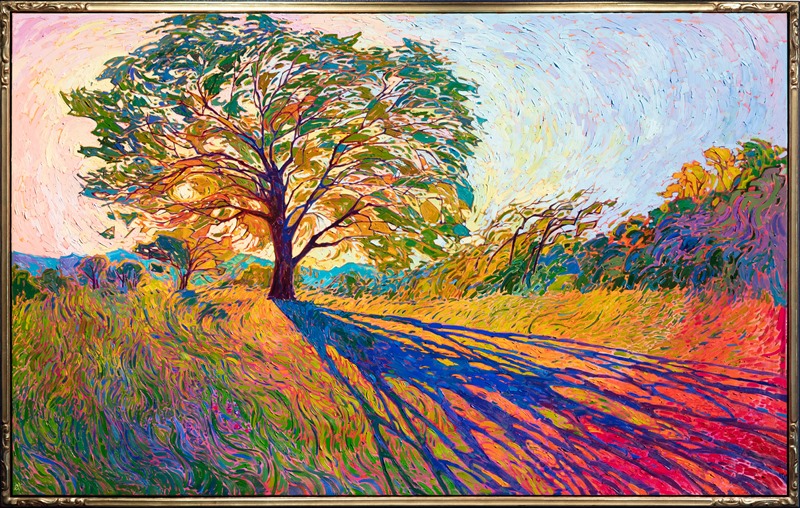This image captures an artwork in a rectangular landscape orientation framed by a thin golden border. The main focus of the art is a large, prominent tree situated slightly to the left of center, with a thick brown trunk and a vibrant canopy predominantly green with accents of yellow and orange. Surrounding the tree is a shadow in a deep blue hue extending towards the bottom right of the canvas, augmenting the complex interplay of colors. The background features a sky with swirling patterns, transitioning from a peach color on the top left to a bluish tone on the top right, evocative of a Van Gogh style. The ground beneath the tree and around the canvas is richly colored with swirling grass and other smaller, less prominent trees and bushes, completing the dynamic and visually engaging composition.